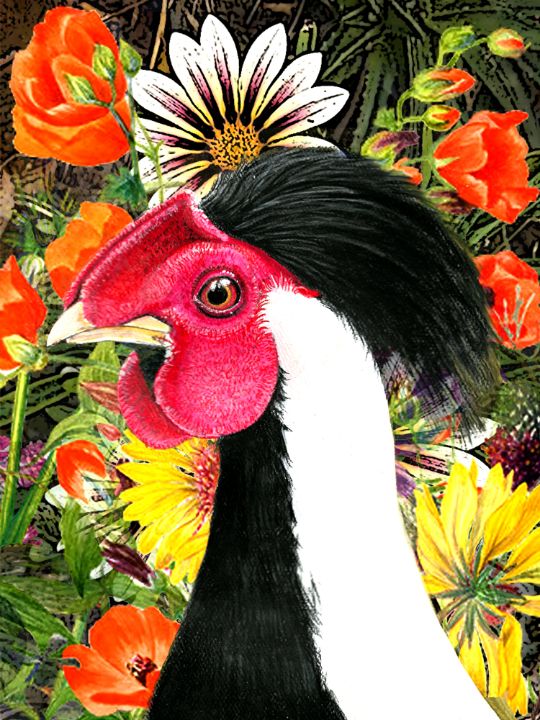This image showcases a highly detailed, handmade painting or a finely penciled portrait of what appears to be a rooster or possibly a vulture. The bird features a unique and striking appearance, with a long snood hanging from the sides of its beak and a bold coloration that splits its neck—black on one side and white on the other. This division of color continues with black feathers curling from atop its head and cascading down towards the right, almost resembling long human hair. Its face displays vibrant red skin flaps reminiscent of turkey markings, while its beak is an off-white shade, becoming more white at the tip. The bird is positioned in front of a backdrop of flowers, rendered in a less realistic yet still vivid style. The flowers include a variety of colors like orange, yellow, white, and purple, with identifiable types such as tulips and daisies, which enhance the contrast and beauty of the bird's striking appearance.